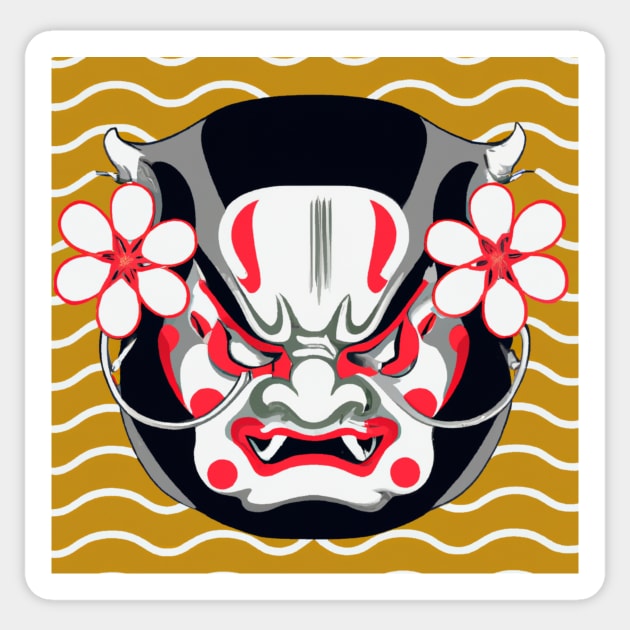This vibrant image showcases a striking artwork resembling a dragon-like mask with pronounced Asian influences. The mask features a predominantly black and gray color scheme with vivid red accents highlighting its intense expression. Red lines frame the slanted, fierce eyes, and deeply accentuate the mouth and cheekbones, adding to its ferocious appearance. The mask displays an intricate pattern of red dots: four on the cheeks — two at the top and two towards the bottom chin. The forehead boasts red lines that extend from the eyes and across the cheeks like stems, culminating in red-outlined flowers with white petals. Sharp fangs peer out from the mouth, enhancing its formidable look. The mask also has small, pointy horns on either side, adding to its mythical allure. The background radiates a warm mustard yellow hue interspersed with wavy white lines, contrasting the dark and rich colors of the mask. Red-outlined flowers with white petals and red star-like centers are situated where ears might be, completing the piece's evocative and detailed visual impact.